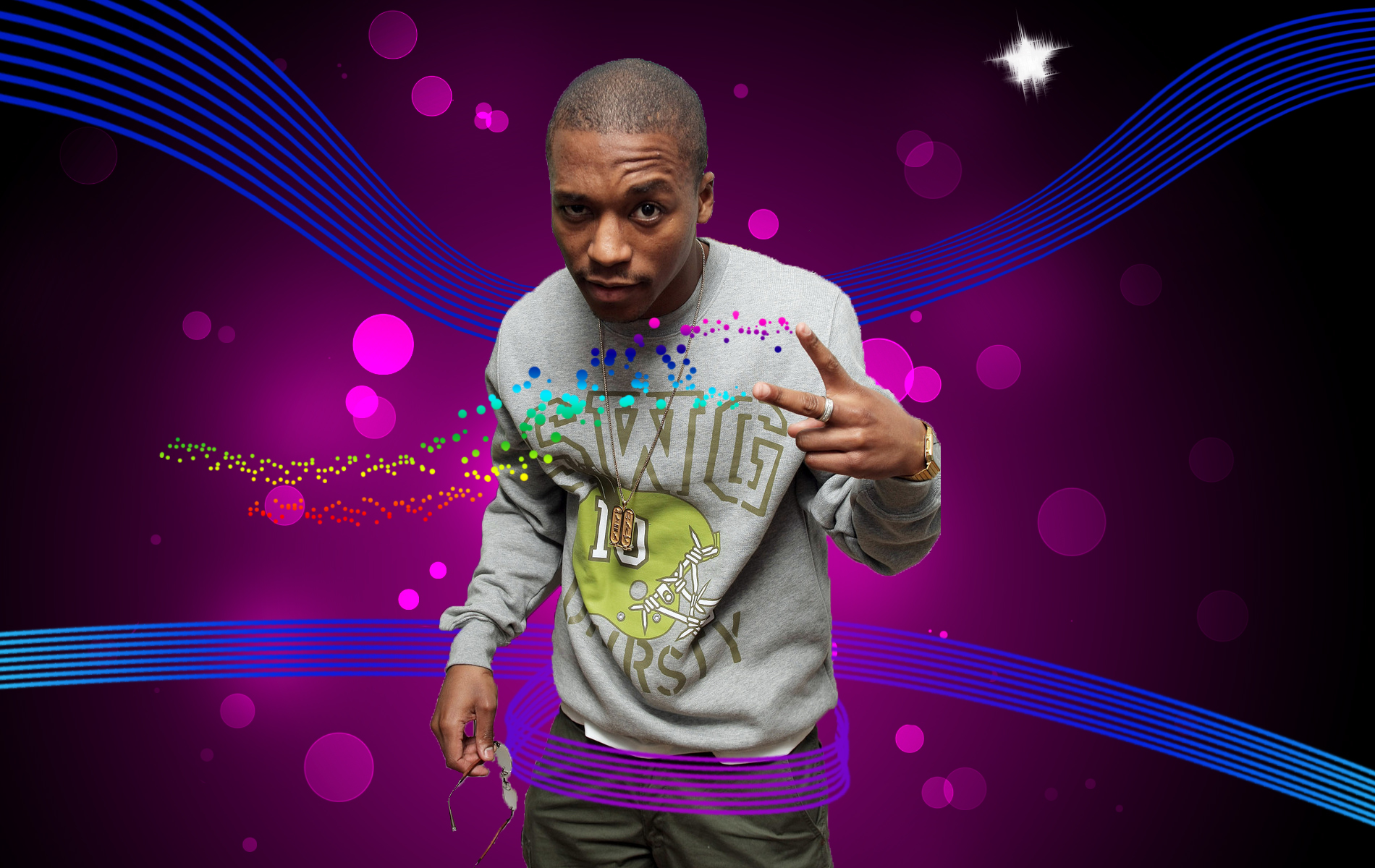The image features a young African-American man in his mid-20s to early 30s, standing against an artistically enhanced, digitally manipulated background. He has short black hair and is raising his right eyebrow, creating noticeable wrinkles above it. Dressed in a gray sweatshirt with "SWG" and a partial "RSTY" visible on it, he appears to embody a confident, possibly creative figure such as a musician or actor.

On his right hand, he's making a sideways peace sign, his middle finger adorned with a silver ring. His left hand holds sunglasses. He's also wearing baggy green pants. The background is a rich dark purple, filled with numerous artistic elements like blurry circles and sparkles. Prominent blue, wavy lines crisscross the scene, flowing from his shoulder and waist and resembling musical instrument strings. Around his midsection, these lines form a loop, wrapping around him and contributing to the vivid, almost ethereal atmosphere. Towards the top right of the image, a single blurry white star adds to the layered visual intrigue of the composition.